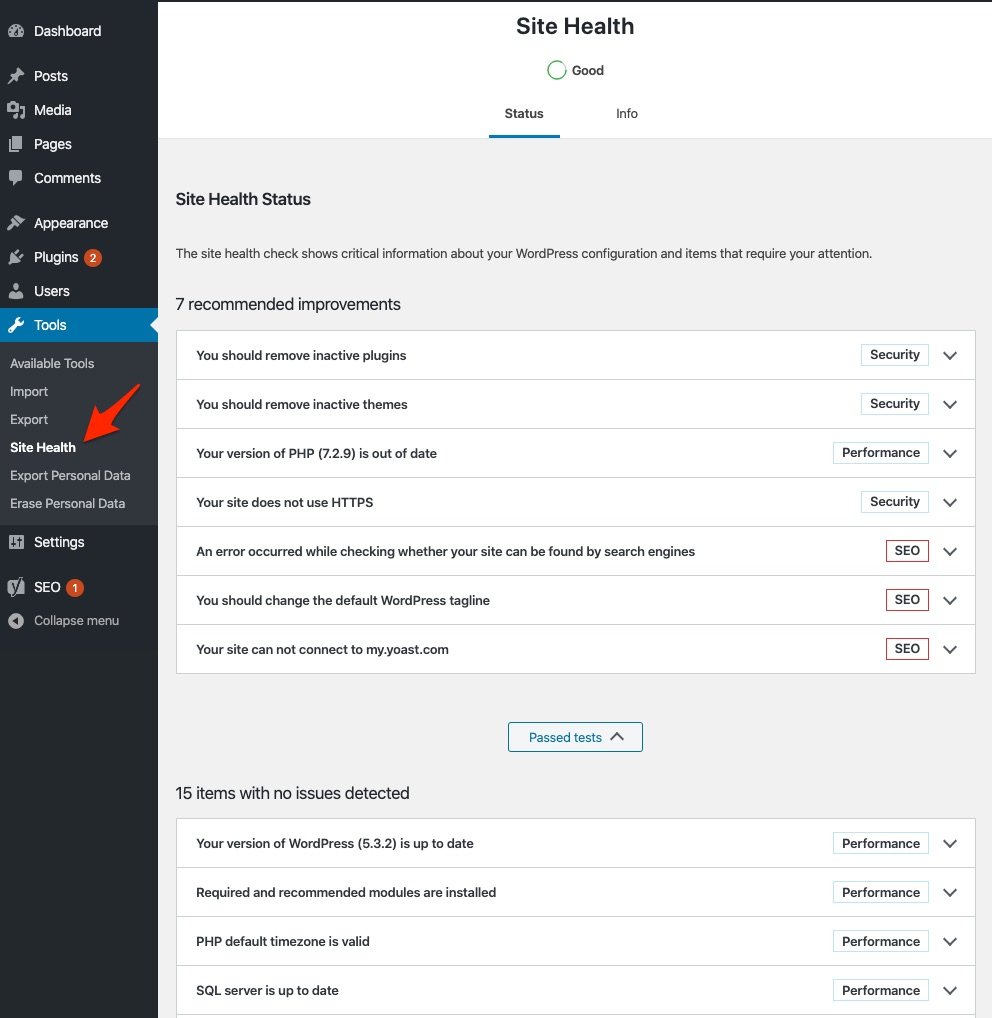A screenshot from a WordPress dashboard highlighting the 'Site Health' section. On the left, a vertical black sidebar features an array of navigation options with text and occasional icons, including 'Dashboard,' 'Posts,' 'Media,' 'Pages,' 'Comments,' and 'Appearance,' among others. Notably, the 'Plugins' section has a red circle with the number two, indicating updates or alerts. The main area of the screen is white to grayish, with a focus on the 'Site Health' status, which is marked as 'Good.' The status section is underlined, leading to detailed information that mentions, "The site health check shows critical information about your WordPress configuration and items that require your attention." It also highlights seven recommended improvements and a 'Past Test' area showing 15 items with no issues detected.